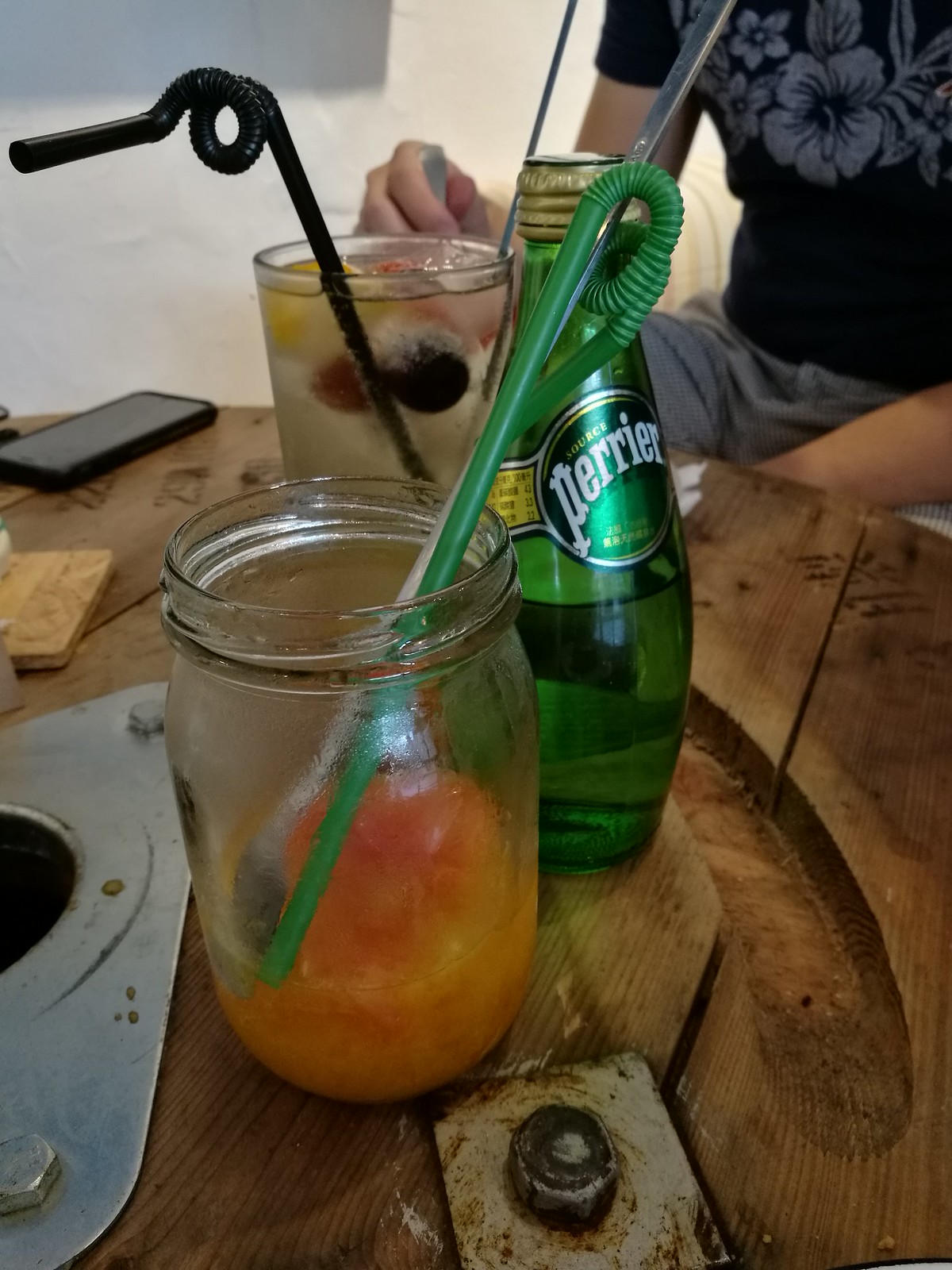The image shows a round wooden table with a reddish-brown finish and several noticeable features, including a half-circle hole on the right side and metal hardware that is scratched and dented. The table is topped with three distinct glass containers. In the foreground is a mason jar containing a red liquid and a gray substance, with one green and one transparent straw sticking out of it. Positioned behind this jar is a green bottle labeled "Perrier" with a brown cap, partially filled with liquid. Further back is a tall, clear glass filled with a cloudy white substance and assorted red, black, and yellow particles, possibly fruits or berries, stirred by a black straw that has a circular top. In the top right corner of the image, a person wearing a black shirt with a floral design and gray trousers or shorts is partially visible. On the far left of the table, there is a black cell phone with its screen turned off. The table’s background area appears to be white, suggesting an indoor or patio setting.